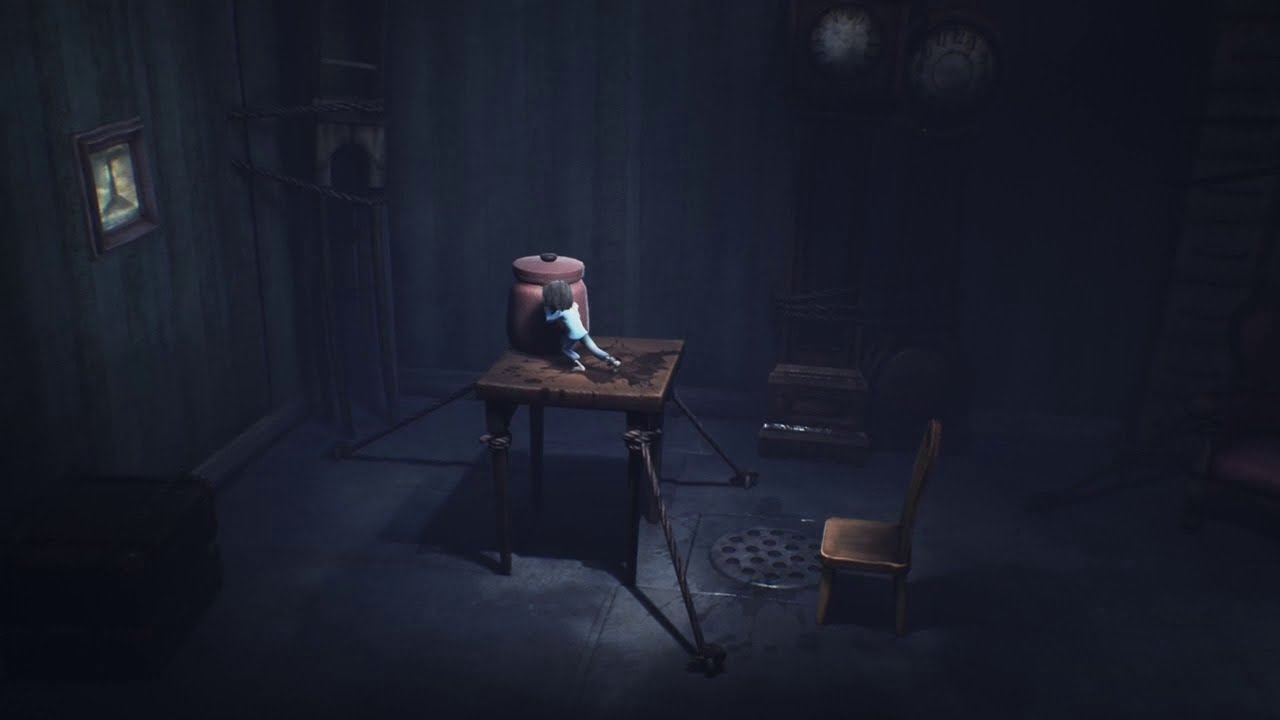In this computer-generated image resembling a scene from a video game, a very dark and dingy room is depicted with a rustic, shadowy ambiance. Central to the room is a wooden table, intricately tethered to the floor by ropes. On this table stands a small character, possibly a girl with long hair, clad in light-colored clothing and leaning against a large red cookie jar. Adjacent to the table, there's a small wooden chair and a manhole cover or drain embedded in the wooden floor. 

The room's perimeter is cluttered with various shadowy outlines, including two distinct grandfather clocks—one fully structured and another skeletal—in different corners, both bound by ropes. A wooden chest and some unidentified items are propped up along the edges, contributing to the room’s eerie atmosphere. The left wall bears a framed picture that seems to depict a tower, adding to the overall sense of mystery. The dim lighting accentuates the central table and its unusual scene, leaving the rest of the room engulfed in shadow.